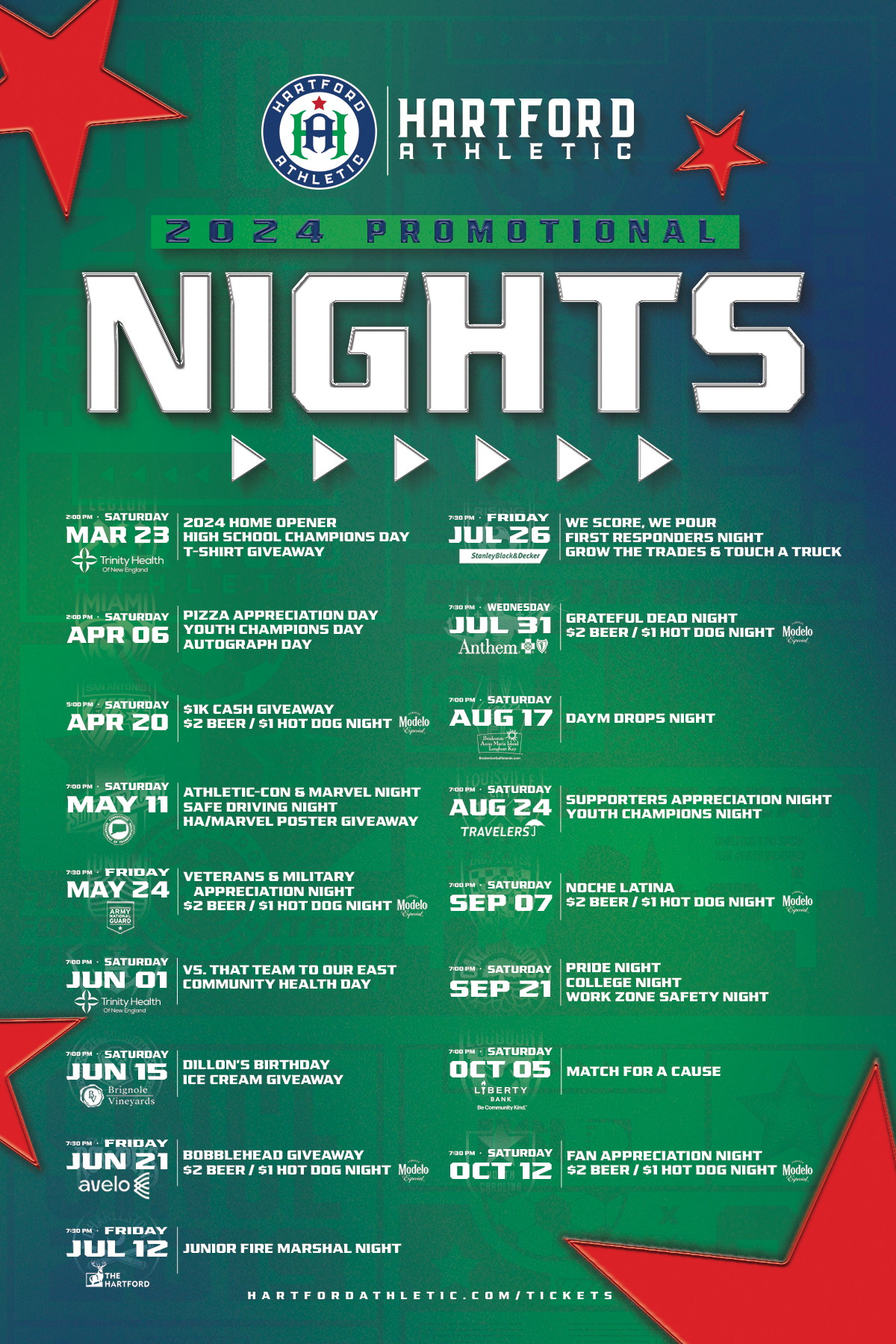This is a detailed 2024 promotional schedule poster for the Hartford Athletic, presented on a blue and green gradient background. At the top, it features the Hartford Athletic logo—a blue, circular emblem with the text "Hartford Athletic" around a white circle containing a green 'H' and a blue 'A'. Alongside the logo, "Hartford Athletic" is written in bold white lettering, accompanied by a red star to its right. Beneath this, a green bar with blue text announces "2024 Promotional", followed by "Knights" in large white letters. Directly below, six white arrowheads point to the right.

The calendar itself is organized in two columns, with events spanning from March 23rd to October 12th. Key highlight dates include:

- **Saturday, March 23rd:** 2024 Home Opener, High School Champions Day, T-shirt Giveaway.
- **Saturday, April 6th:** Pizza Appreciation Day, Youth Champions Day, Autograph Day.
- **Friday, May 24th:** Veterans and Military Appreciation Night, $2 beer, $1 hot dog night.
- **Saturday, June 1st:** Versus That Team to Our East, Community Health Day.
- **Saturday, June 15th:** Dylan's Birthday, Ice Cream Giveaway.
- **Friday, June 21st:** Bobblehead Giveaway, $2 beer, $1 hot dog night.
- **Friday, July 26th:** We Score, We Pour, First Responders Night, Grow the Trades, Touch a Truck.
- **Saturday, August 17th:** Day M Drops Night.
- **Saturday, September 21st:** Pride Night, College Night, Work Zone Safety Night.
- **Saturday, October 12th:** Fan Appreciation Night, $2 beer, $1 hot dog night.

Each date features specific events and giveaways such as T-shirts, posters, and themed nights like Marvel Night and Grateful Dead Night. The bottom of the poster lists HartfordAthletic.com/tickets for more information. Red stars of varying sizes are interspersed throughout the design, adding vibrant highlights to the overall aesthetic.